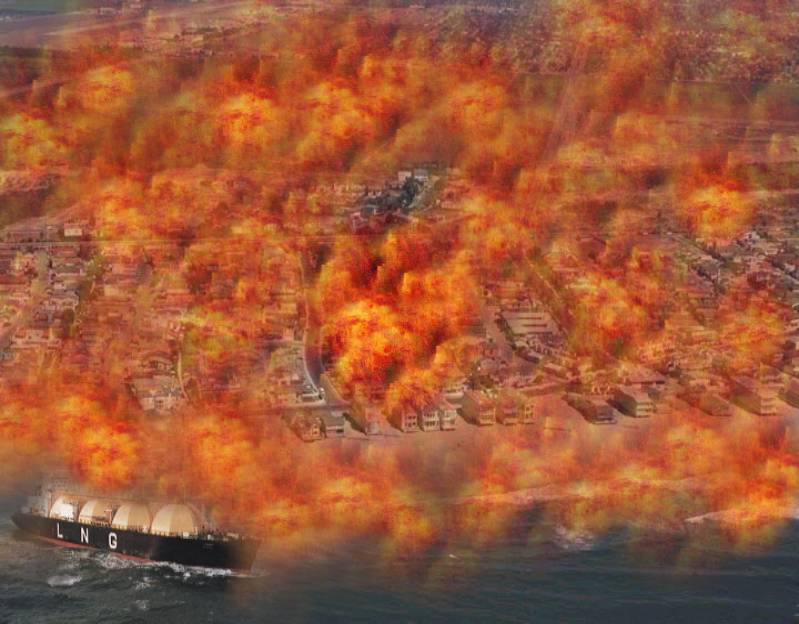This image depicts a dramatic scene of a city or town on fire along a shoreline, rendered in various shades of orange, red, and yellow. The vivid, almost surreal flames blend with dark gray smoke, creating an impression of chaos and destruction. In the bottom left corner, a black vessel with white lettering that reads "LNG" is visible, adorned with four white dome-shaped structures on its deck. The ship appears small against the vast, fiery backdrop. The water near the ship is a dark blue, contrasting with the fiery hues dominating the scene. The fire engulfs most of the image, highlighting the devastation, while faint outlines of buildings can be discerned through the intense, glowing clouds.